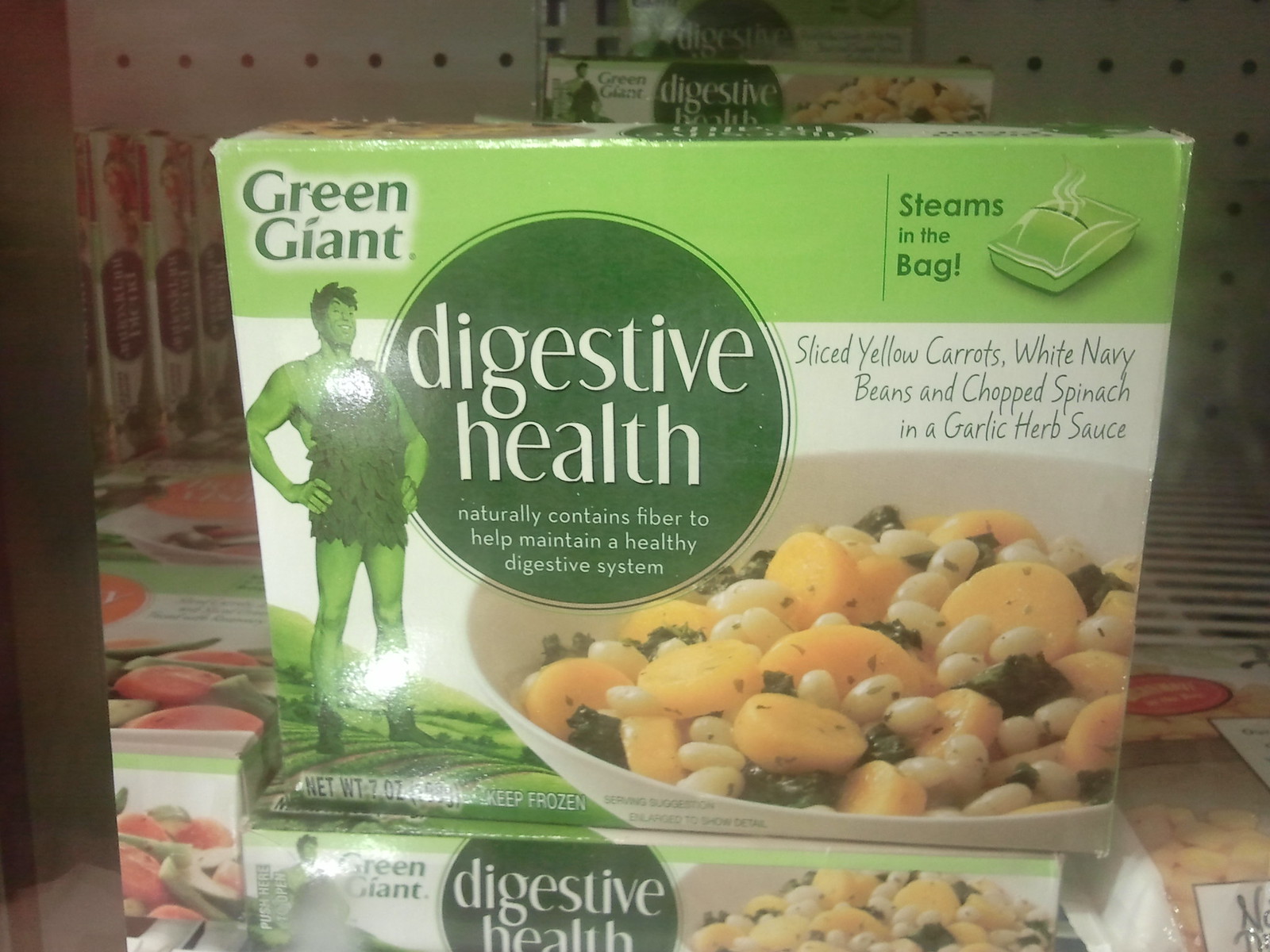This horizontal rectangular photograph, taken in a supermarket or convenience store, captures several stacked packages of Green Giant's "Digestive Health" steams-in-the-bag meal. The focal point is a green and white box prominently featuring the Green Giant logo in green font on a white background in the upper left-hand corner. Below the logo, the Green Giant character stands confidently with hands on his hips, dressed in a green toga-like outfit made of leaves. To his right, a large, dark green circle with a lighter green center contains white, bolded text reading "digestive health." Beneath this, in smaller white font, are the words "naturally contains fiber to help maintain a healthy digestive system."

Central to the package is an appealing image of the meal: a white plate filled with sliced yellow carrots, white navy beans, and chopped spinach, all enveloped in a garlic herb sauce. The background includes other product boxes and a white pegboard, adding depth to the scene. The overall design effectively emphasizes the product's health benefits and enticing food presentation.